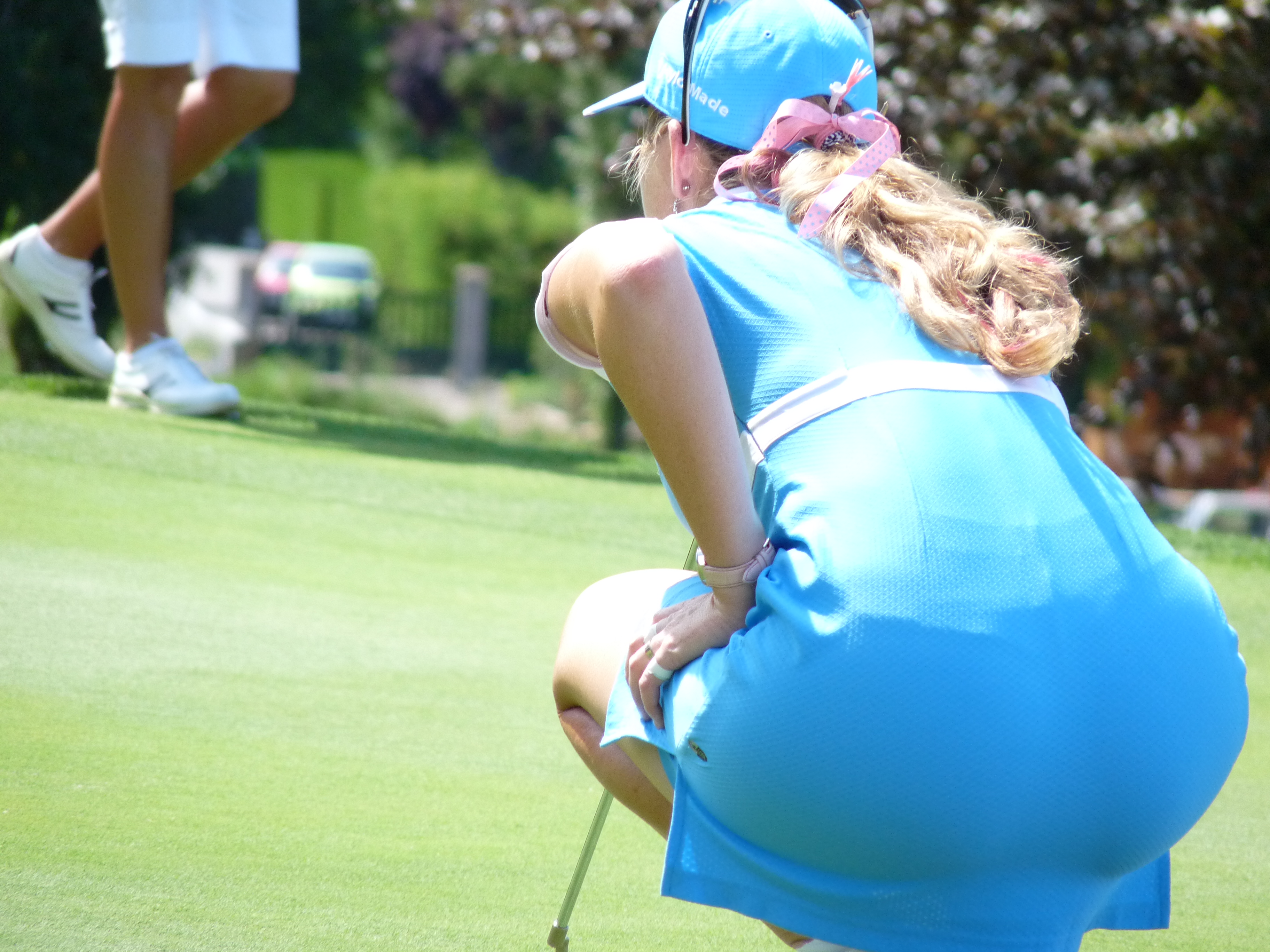This is a photograph of a woman golfer lined up to putt on a vibrant green golf course. The course slopes downwards from the upper left to the bottom right of the wide rectangular frame. The woman, dressed in a light blue dress adorned with a pink belt and pink sleeves, is kneeling with her back to the camera on the lower right side of the image. She wears a blue cap with white text, accented by a pink bow over her long blonde curly hair that drapes down her back. Sunglasses rest atop her cap. Her left elbow is bent with her hand resting on her left thigh, which is bent and partially visible beside her dress. Her right hand holds a putter that stretches down to the green. In the upper left corner, a person in white shorts and white sneakers is walking downhill, situated near a tree that is visible on the far right. The sky is clear, suggesting it is a sunny day. There is also a bush with purple or lavender flowers above the golfer's right shoulder and some green foliage in the center background. The scene captures a moment of focused concentration as the woman aligns her putt.